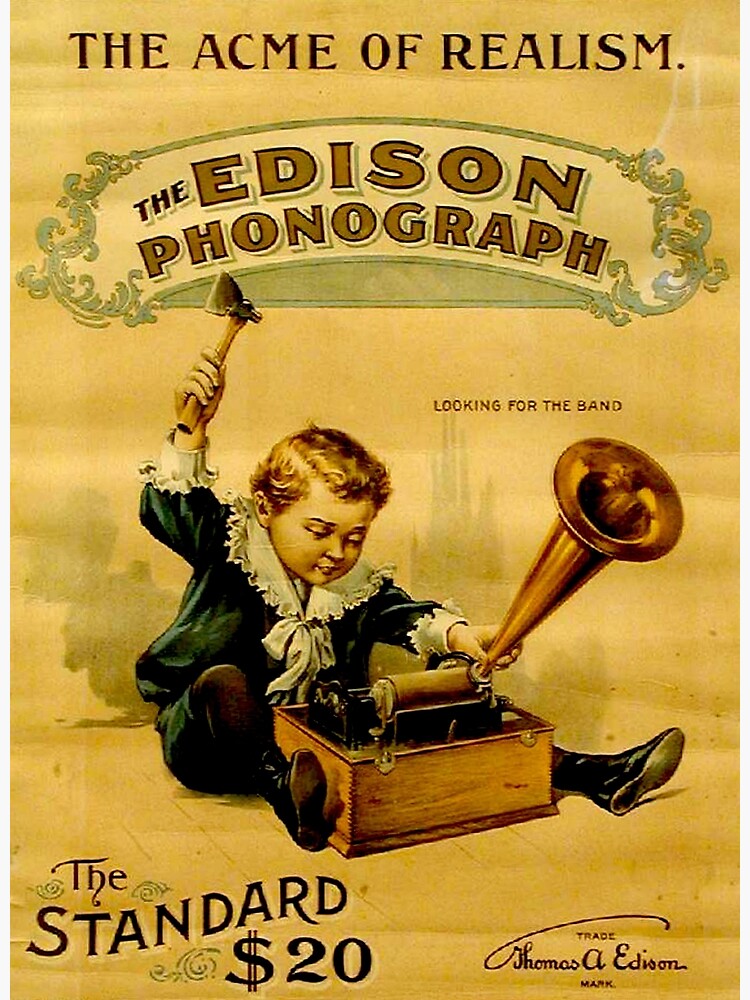This advertisement poster for "The Edison Phonograph" showcases the slogan "The Acme of Realism" at the top. The central image features a small child dressed in antiquated clothing, poised to strike with a tomahawk held high in his right hand. In his left hand, he grasps a large, golden phonograph horn. The scene depicts the child about to destroy the phonograph—a wooden, rectangular device with a roller component—highlighting an unusual and eye-catching approach. The background has a yellow tint, and the shadows of both the child and the horn are visible, adding depth to the imagery. At the bottom, the poster mentions "The Standard $20," and carries the trademark of Thomas A. Edison.